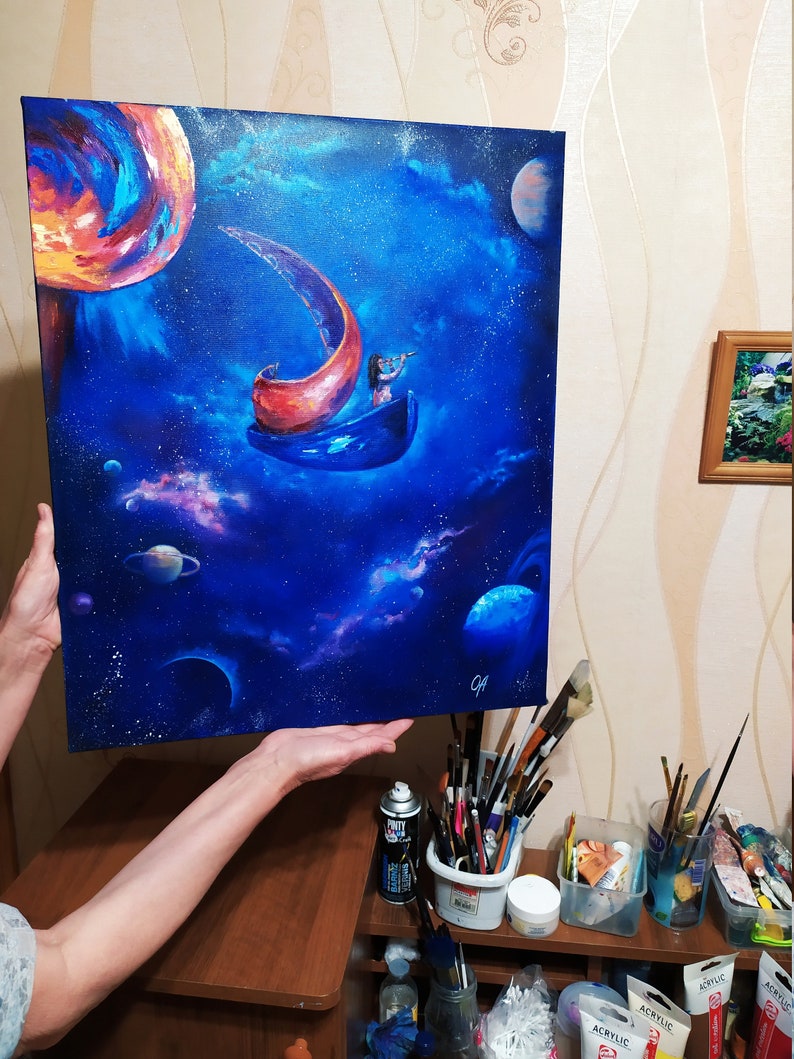In the image, the background features a soft, light brown hue. Emerging from the bottom left corner are a pair of hands, delicately holding a large painting. The artwork, filled with varying shades of blue, vividly depicts a nighttime sky. Central to the composition, a girl with long, dark hair sits in a blue canoe that has a distinctive red stern. She holds a scope, intently gazing into the celestial expanse around her. The backdrop of the painting is adorned with numerous circular planets, scattered across the scene. Particularly striking is the large planet in the upper left corner, which is an explosion of colors – blue, red, orange, and yellow. Adjacent to this vivid portrayal, to the right, a shelf brims with artistic tools. The top shelf holds several containers bristling with long paintbrushes and other art implements, while below, numerous plastic containers house an array of vibrant paints.